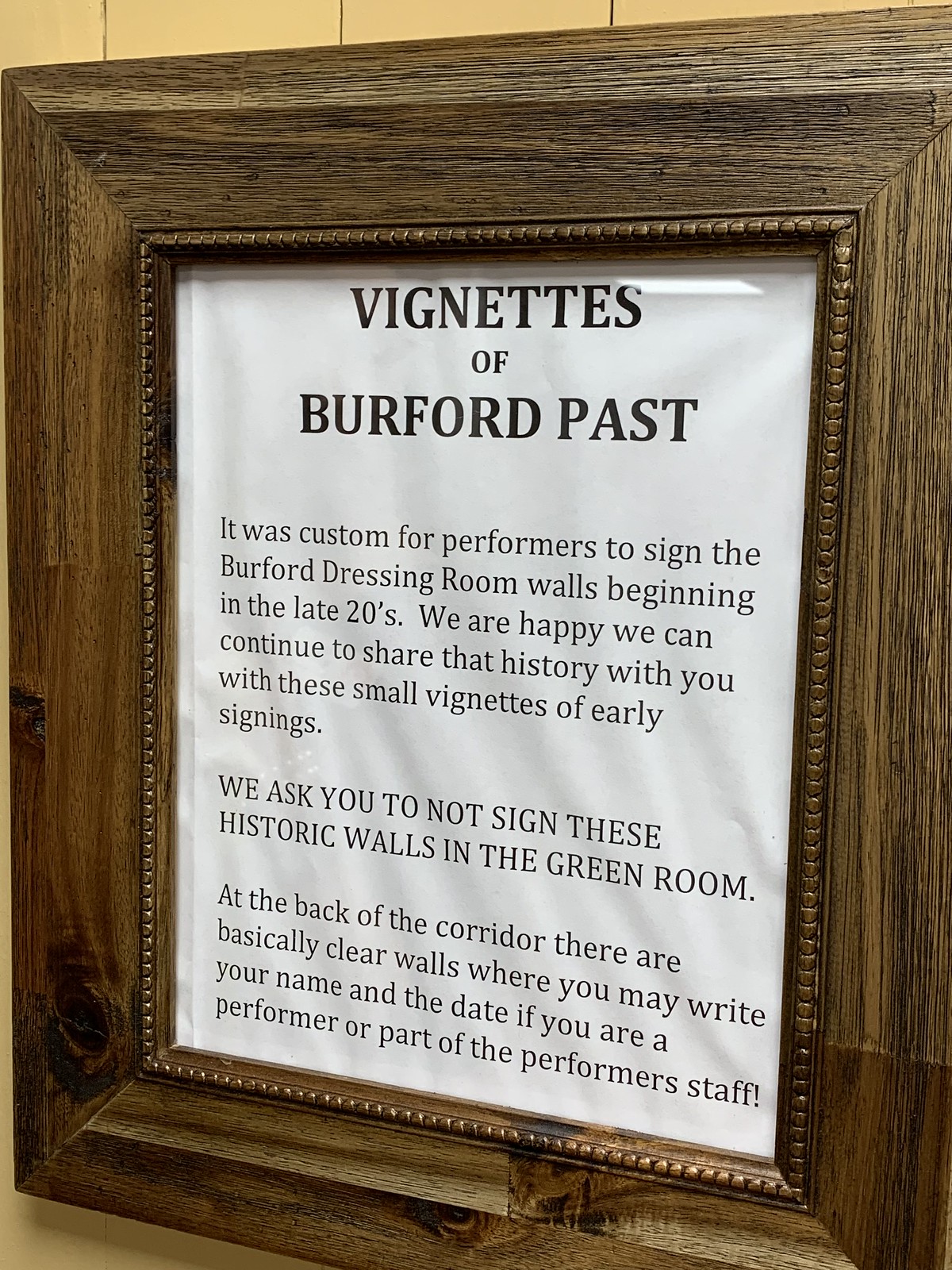A wooden picture frame adorns a wall, enclosing a piece of paper with black lettering. At the top of the paper, a prominent heading reads, "Vignettes of Burford Past." Below the heading, in smaller font, the text provides a glimpse into the historical tradition: "It was custom for performers to sign the Burford dressing room walls beginning in the late 20s. We are happy we can continue to share that history with you, with these small vignettes of early signings. We ask you to not sign these historic walls in the green room. At the back of the corridor, there are clear walls where you may write your name and the date if you are a performer or part of the performer's staff." The frame not only captures historical anecdotes but also respectfully maintains the venue’s legacy by guiding contemporary performers on where they can leave their marks.